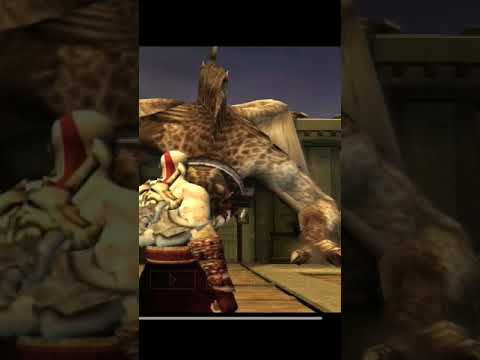The image appears to be a snapshot from a God of War video game, characterized by its digital art style. The scene is depicted within a square frame, with a highlighted vertical rectangle in the center, emphasizing the main action. In both the background and the highlighted area, there is a large, brown-tan, dragon-like creature with wings, set against a blue sky and a building. The protagonist, standing upright with his back towards the viewer, is positioned at the lower left corner of the vertical rectangle. He is facing the dragon, which is towards the top left of the frame. The character is notably muscular, possibly adorned with tattoos, and wears either a red skirt, kilt, or baggy pants. A distinctive red stripe is painted across his head. He also appears to have a sword sheathed on his back, indicating readiness for battle. The image has a slightly pixelated, low-quality appearance, suggesting it may be from an older console, possibly one of the early PlayStation systems. The primary colors in the scene include shades of white, red, black, brown, beige, dark blue, and gray.